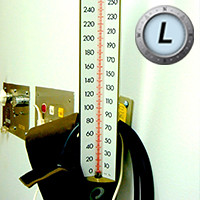In this image, we see a closely framed photograph of a blood pressure cuff. The cuff connects to a gauge displaying measurements from 0 to 250, incremented by tens (0, 10, 20, 30, 40, 50, etc.), though the upper portion of the gauge is cut off. Attached to the cuff is a pewter-colored round medallion with a white button in the center bearing the letter "L". In the background, a dull white wall is adorned with several small photographs affixed using tape or thumbtacks. Among these, one photo stands out, depicting a child walking on a path, though the remaining images are indistinct. The overall atmosphere suggests a clinical or home health monitoring setting.